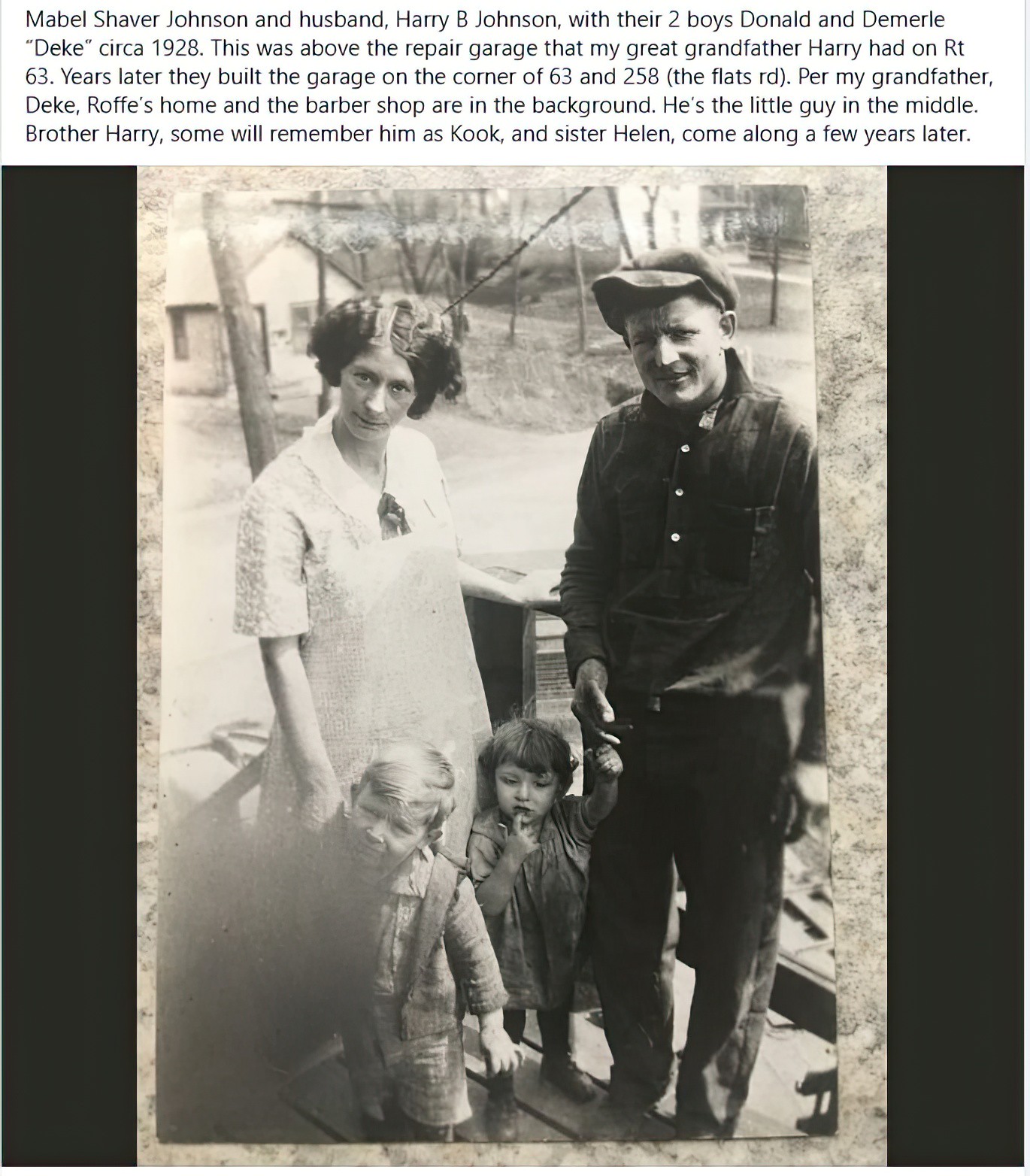A black and white photograph from circa 1928 depicts Mabel Shaver Johnson and her husband Harry B. Johnson standing with their two young sons, Donald and Demerle "Deke." Mabel, wearing a light-colored dress, holds the hand of one child while Harry, dressed in dark clothing and a floppy cap, holds the hand of the other. The children are dressed in grayish attire and stand between their parents on what appears to be a wooden deck. The setting is outdoors, likely during the day, with a couple of houses visible in the background. The caption above the photo reads, "Mabel Shaver Johnson and husband Harry B. Johnson with their two boys Donald and Demerle Deke, circa 1928." This image was taken above the repair garage that Harry owned on Route 63, with later mention of a garage on the corner of Route 63 and Flats Road built for their son, Deke.